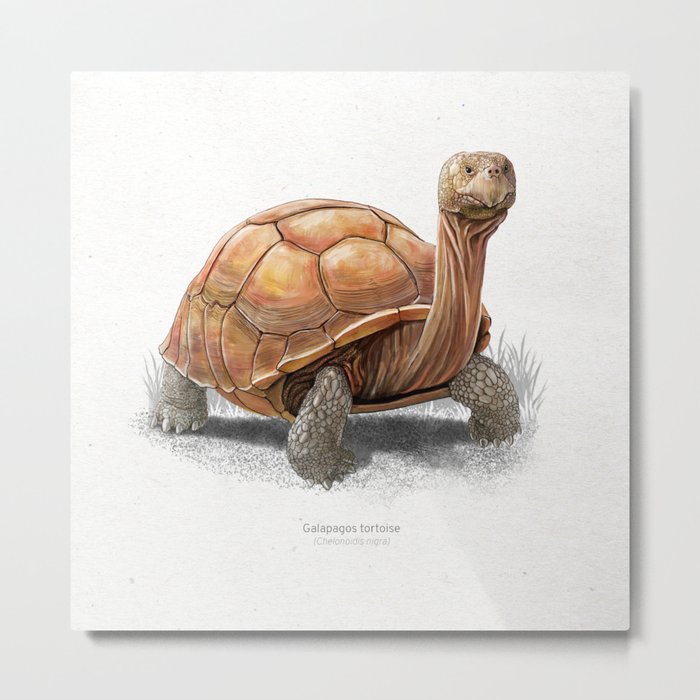This is a detailed illustration of a Galapagos tortoise, rendered in colored pencils. The drawing is centered on a white background, likely an art pad or a sketch board. The text below the tortoise reads "Galapagos tortoise Chelidonis nigra" in very light gray letters. The tortoise occupies the central part of the image, with its head facing the bottom right corner. Its front legs are turned inward, showcasing their gray, leathery texture with prominent scales and bumps. The head, characterized by a hard, leathery pattern similar to the legs, features a pointy nose resembling a beak, tiny nostrils, and black eyes. The neck appears wrinkled and tan, indicating loose skin. The shell is large, rounded, and colored in shades of light tan, brown, and pinkish-orange, with distinctive plates. This image, resembling a nature guide style, provides a comprehensive and realistic view of this majestic reptile.